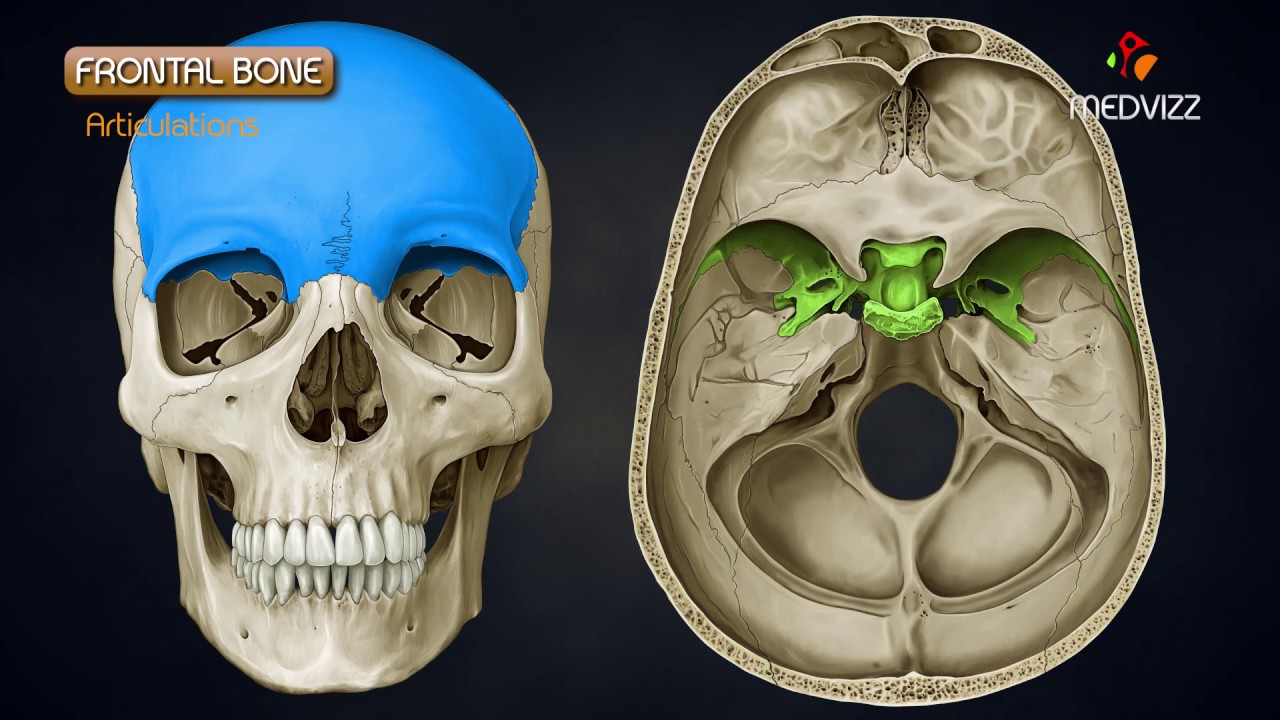The image features a detailed digital representation of the frontal bone of a human skull against a dark blue background. On the left side, a forward-facing view of a skull is presented, wherein the frontal bone is distinctly highlighted in bright blue. The rest of the skull is displayed in a light beige or bone-white color. Directly beneath the brown caption labeled "Frontal Bone" in white letters, the term "Articulations" is written in brown letters. Conversely, the right side of the image shows a cross-sectional top view of the skull, emphasizing the internal structure, with a section in front of the opening for the spinal column marked in green. An orange, green, and red logo labeled "MEDVIZ" is positioned in the upper right corner. The skull illustration includes detailed features such as eye sockets, the nasal cavity, and teeth, presenting a comprehensive anatomical view.